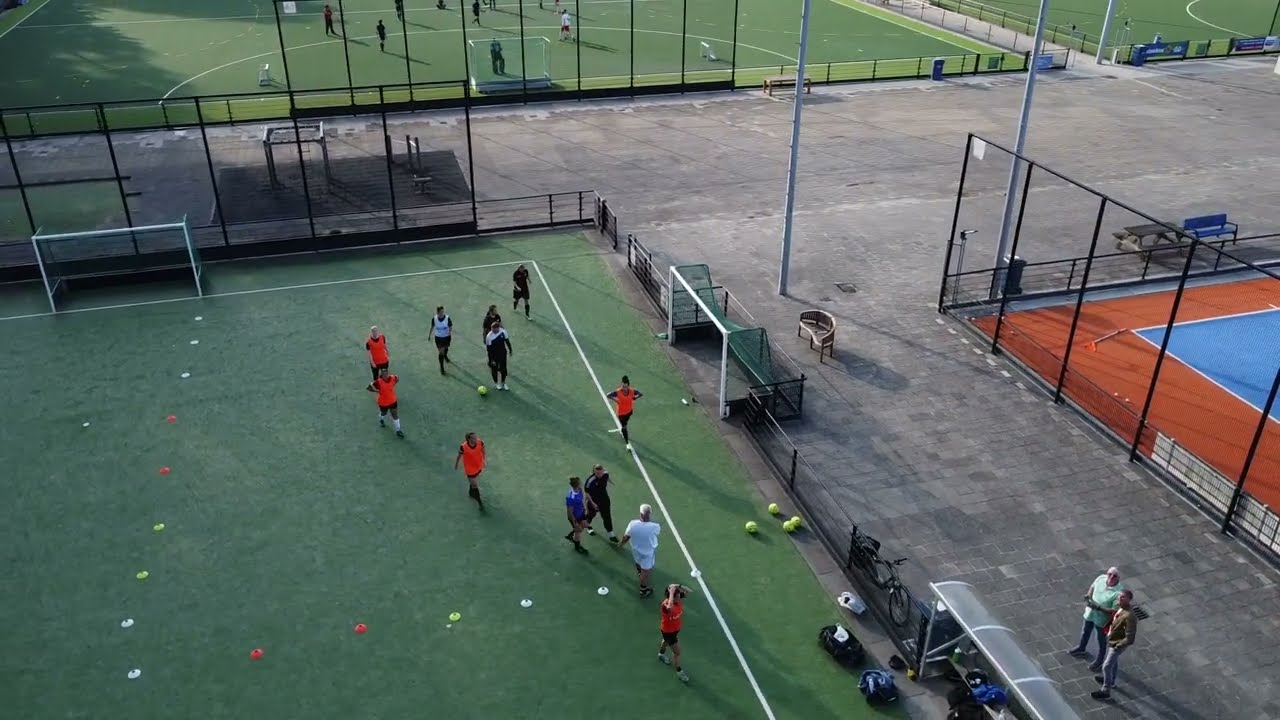This image, taken from an overhead drone perspective around 100 feet high, depicts a multi-field outdoor sports complex in daylight. The main focus is a women's soccer practice on a green artificial turf field located towards the bottom left. Approximately ten players are visible, with some wearing orange and black jerseys while others don white and black. Various training equipment, including balls and cones, is scattered across the field. Two grown men, presumably coaches, observe the activity from a nearby concrete walkway.

To the top of the image, there is a larger soccer field, possibly regulation size, hosting another team dressed in dark colors. This field also appears active with several players engaged in practice. Additionally, on the right side of the image—more towards the bottom—a tennis court can be seen. It has a distinct brown border and a blue playing surface.

The landscape-oriented photograph, rich in shades of green, light green, red, black, gray, orange, and blue, captures a bustling public sports area, indicating a vibrant and active community space dedicated to athletic activities.